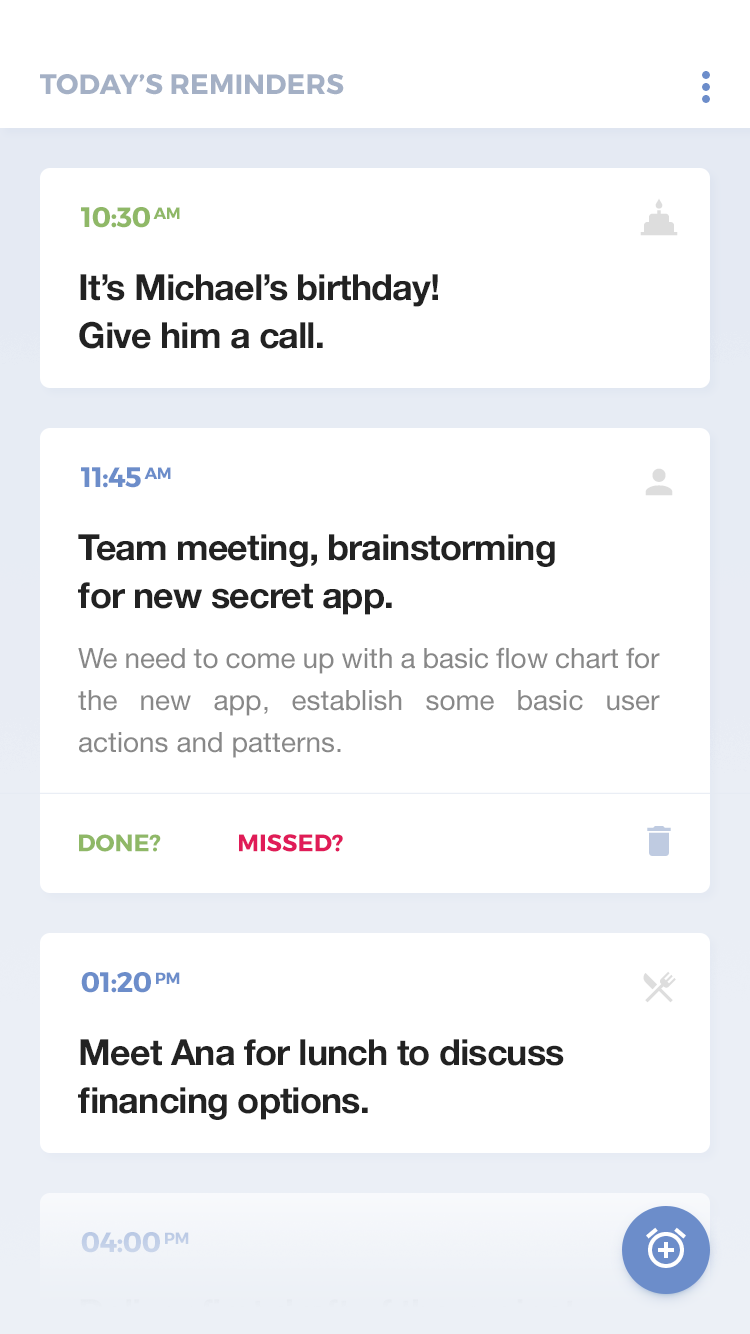The image is a detailed digital reminder list for a specific day, organized within a grayish-blue rectangular interface. At the top, the heading "Today's Reminders" appears in a faint gray color. Adjacent to the text are three vertically aligned circles.

Within a white square on this digital reminder interface, the first reminder states "10:30 a.m." in green text. Directly below, in bold black text, it notes "Michael's birthday - give him a call." In the upper right-hand corner of this section, there's a gray birthday cake icon.

Below that, another reminder on a white background shows "11:45 a.m." in blue text. Beneath it, in bold black text, the task "Team meeting - brainstorming for a new secret app" is listed, followed by a light gray description detailing, "we need to come up with a basic flowchart for the new app, establish some basic user actions and patterns." To the upper right of this section, a gray icon depicts a person's head and shoulders. At the bottom of this reminder box, the words "DONE?" in green and "MISSED?" in red, both in capital letters with question marks, are present. A gray garbage can icon is also included for deleting the reminder.

Further down, against another white background, the reminder indicates "1:20 p.m." in blue text. Below it, in bold black letters, the task "Meet Anna for lunch to discuss financing options" is specified. In the upper right-hand corner, there's a gray icon of a fork and knife.

Lastly, the time "4:00 p.m." is visible in light blue text. To the right, a blue circle contains an old-fashioned white alarm clock icon with a plus sign in the middle. The overall layout is designed to help the user keep track of their daily tasks efficiently.